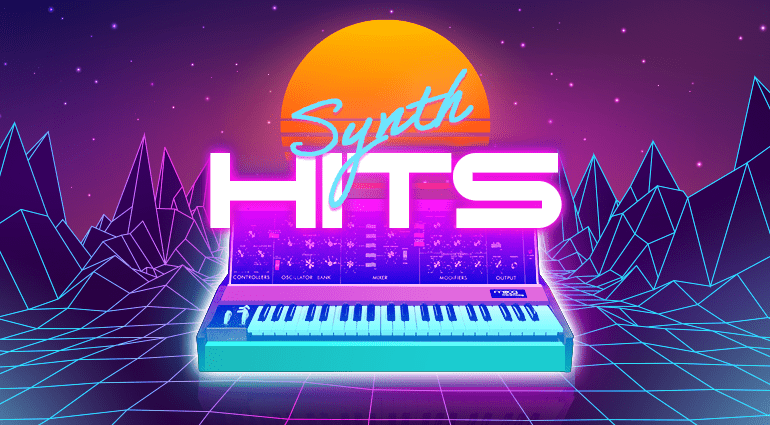The image features an eye-catching, vividly colorful scene that combines elements of both digital and retro aesthetics. The backdrop is a synthesized, dark purple sky speckled with a few tiny stars, transitioning into a bright pink hue closer to the horizon. Cutting through this electrifying sky are computer-generated, graph-like mountains depicted with angular purple and blue lines, lending a geometrical, futuristic touch to the landscape.

Dominating the center of the image is a striking, bright orange sun, of which about three-quarters is visible. Superimposed over the sun, the word “synth” is elegantly written in a blue cursive font, while the word “hits” is displayed in bold, white block letters against the pink background, drawing immediate attention to the message.

Beneath this text, a vibrant musical keyboard takes center stage, exuding a palette of neon teal, black, and white contrasting keys. The front of the keyboard matches the teal hue of the word "synth." The keyboard appears to have a control panel or display at its back, potentially indicating different functions or key sounds, though details are difficult to discern. This image evokes the feel of a dynamic advertisement for a sound engineering or music production program, with its nostalgic yet modern graphic design and richly saturated colors.